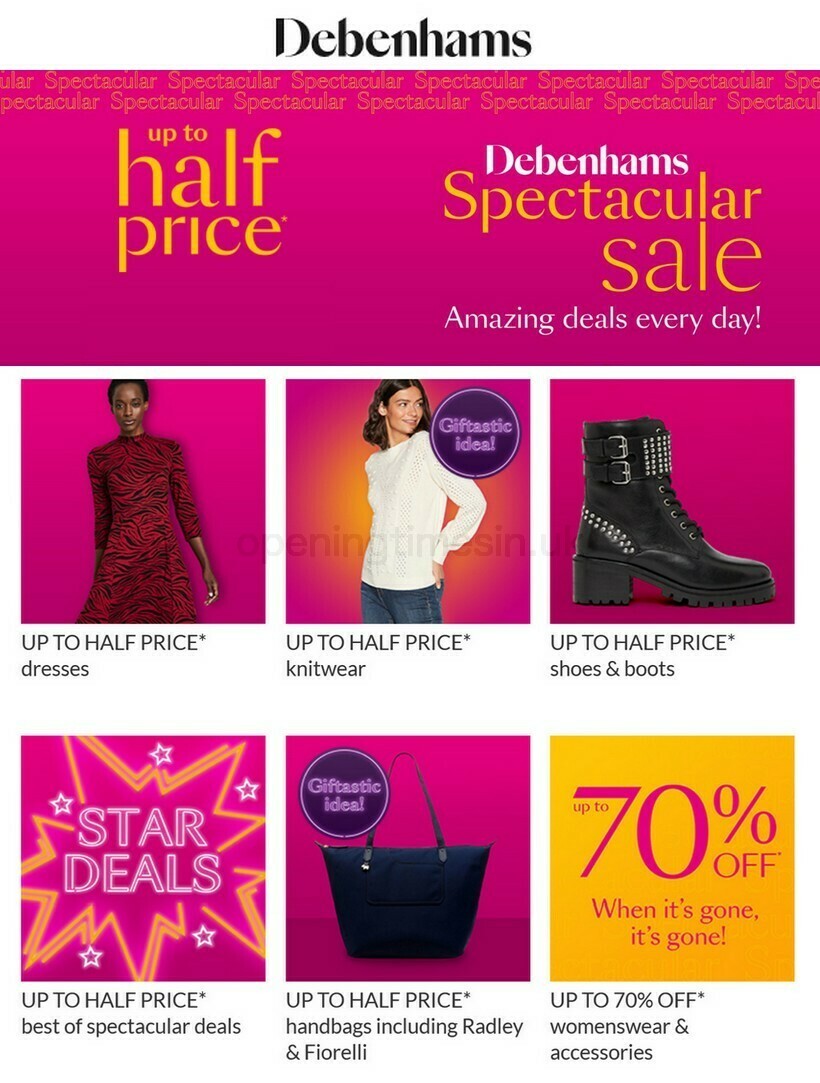The advertisement for Debenhams is visually captivating and meticulously structured to highlight the numerous deals and discounts available. 

At the top of the panel, a crisp white banner prominently features the brand name "Debenhams" in bold black text. Beneath this, a large pink rectangle grabs attention with its dynamic combination of white and yellow lettering. The left side of this rectangle highlights an enticing offer in yellow text: "Up to Half Price." The right side emphasizes the excitement with the text: "Debenhams Spectacular Sale, Amazing Deals Every Day."

Below this main banner are three distinct pink squares, each showcasing a specific product. The first square features a stylish black woman adorned in a chic red and black dress with a caption underneath that reads, "Up to Half Price Dresses." The second square portrays a young girl in a cozy white sweater and jeans. A purple circle with light purple font within this square announces a "Giftastic Ideal." The third square displays a fashionable boot with buckles, accompanied by the caption: "Up to Half Price Shoes and Boots."

Further down, another row of three squares adds to the visual appeal. The first square is pink with a bright yellow star in the center, labeled as "Star Deals." The second square presents a designer handbag set against a pink backdrop, featuring the same "Giftastic Ideal" purple circle. The third square stands out with yellow background and pink lettering, declaring, "Up to 70% Off. When It's Gone, It's Gone."

This Debenhams advertisement efficiently uses vibrant colors and organized sections to clearly convey the variety of sales and special offers, making it an eye-catching and effective promotional display.